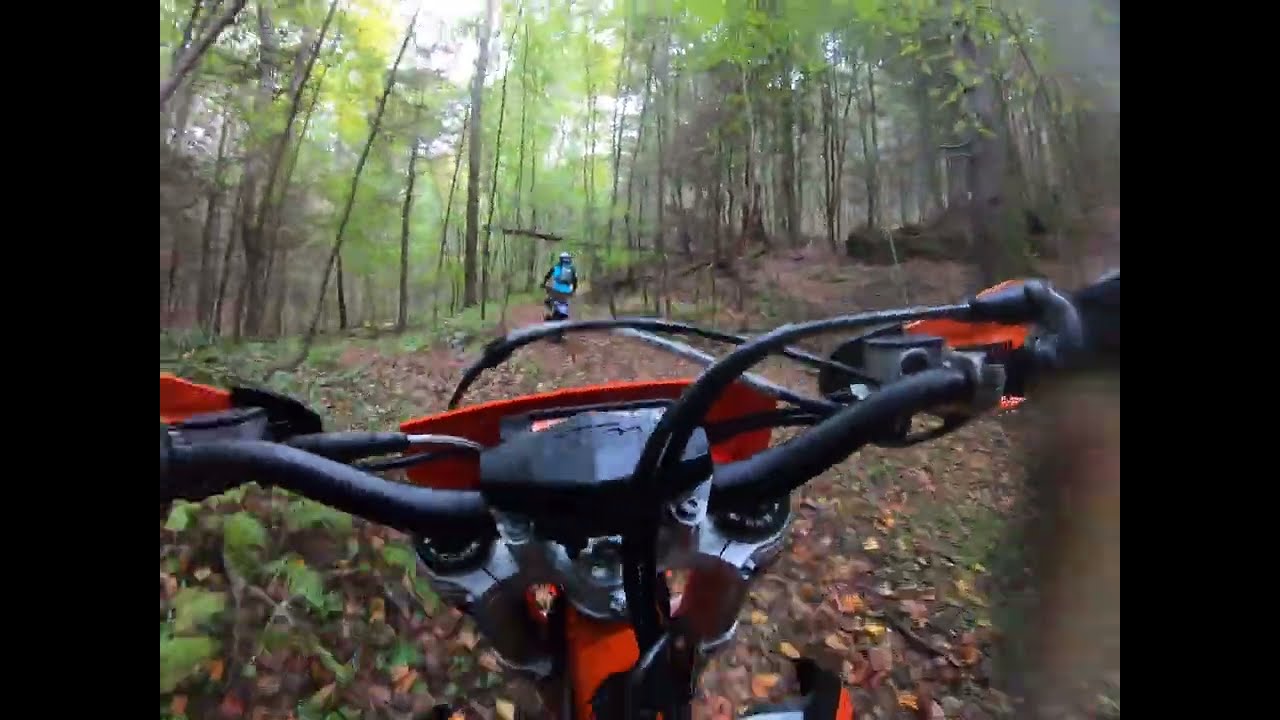The image is a horizontally aligned rectangular photograph framed by vertical black borders on either side, with no borders on the top and bottom. Taken outdoors in a forested area, it depicts a scene from the point of view of a person riding a dirt bike, as seen through a helmet camera. The foreground shows the red and black handlebars of the dirt bike, which stretch across the middle to the bottom of the picture. The hands holding the handlebars are obscured by the black borders. 

Ahead on a leafy and possibly damp path, another biker can be seen wearing a helmet and a blue top, possibly with a backpack. The ground is covered with a mix of yellow and red fallen leaves that stick to the dirt path. Tall, thin-trunked trees with sparse green leaves and numerous branches surround the area, adding to the densely forested atmosphere. The scene also features a slight fog towards the right, suggesting motion as the photograph was taken.